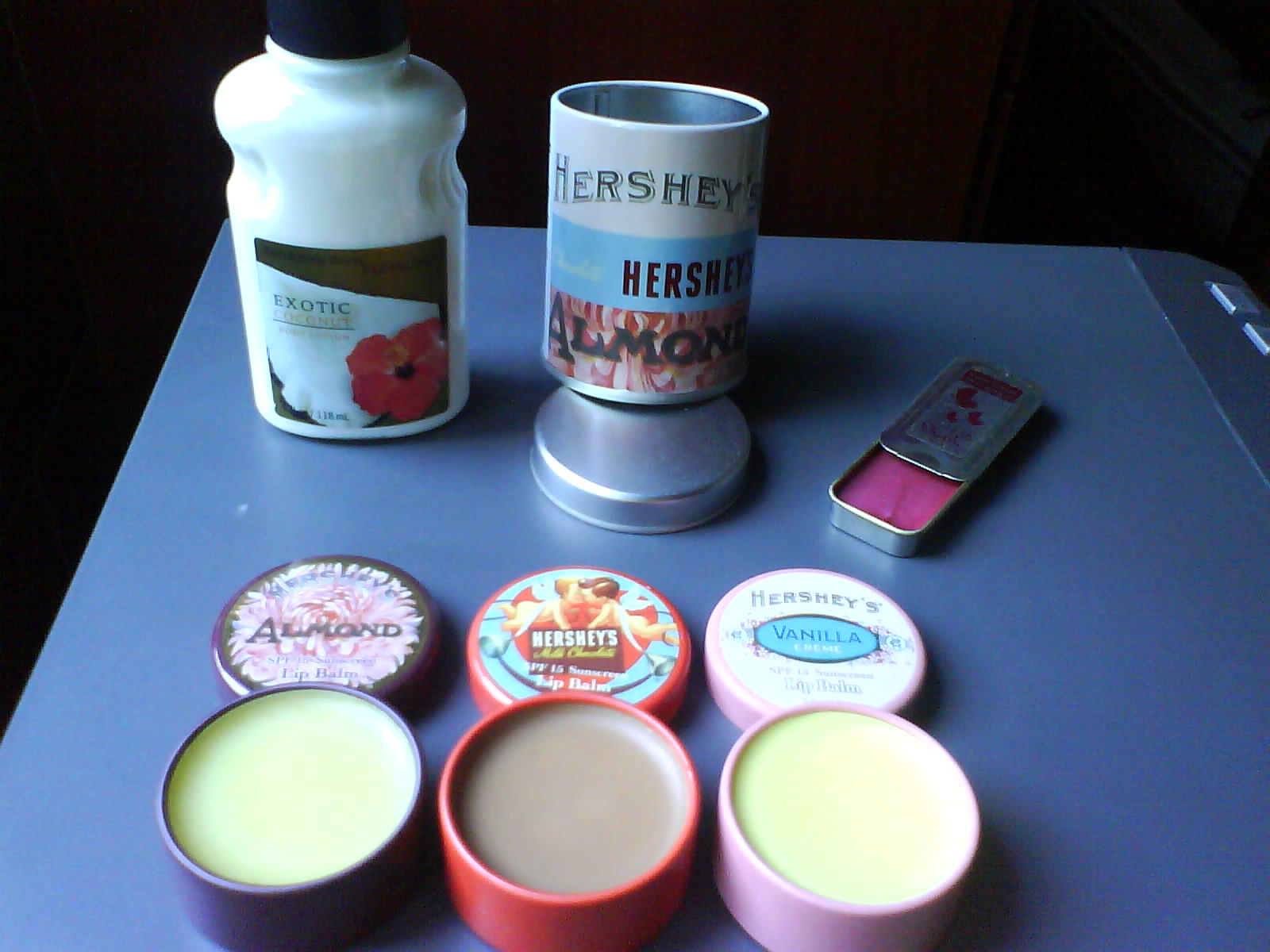This color photograph showcases a meticulously arranged collection of beauty products on a small, square, light blue table. Dominating the top left corner is a tall bottle of white lotion labeled "Exotic Coconut," adorned with a brown label featuring a white coconut piece and a pink flower. Adjacent to this is a short, cylindrical tin with a silver lid, labeled "Hershey's Almond."

At the center sits a slightly open rectangular metal holder revealing a pink balm, possibly Hershey's strawberry-scented. In the front row, a trio of large circular containers with their lids off displays various balms. From left to right: The first container is blue with a yellow balm inside, and its lid, labeled "Almond," rests on top. The middle container, wrapped in red, holds a brown balm with a lid marked "Hershey's." The rightmost container, sporting a pink wrapper, contains a yellow balm and features a lid labeled "Hershey's Vanilla."

This detailed arrangement emphasizes a blend of exotic and familiar, with tropical scents and indulgent Hershey's-themed products, all neatly placed on a light blue platform.